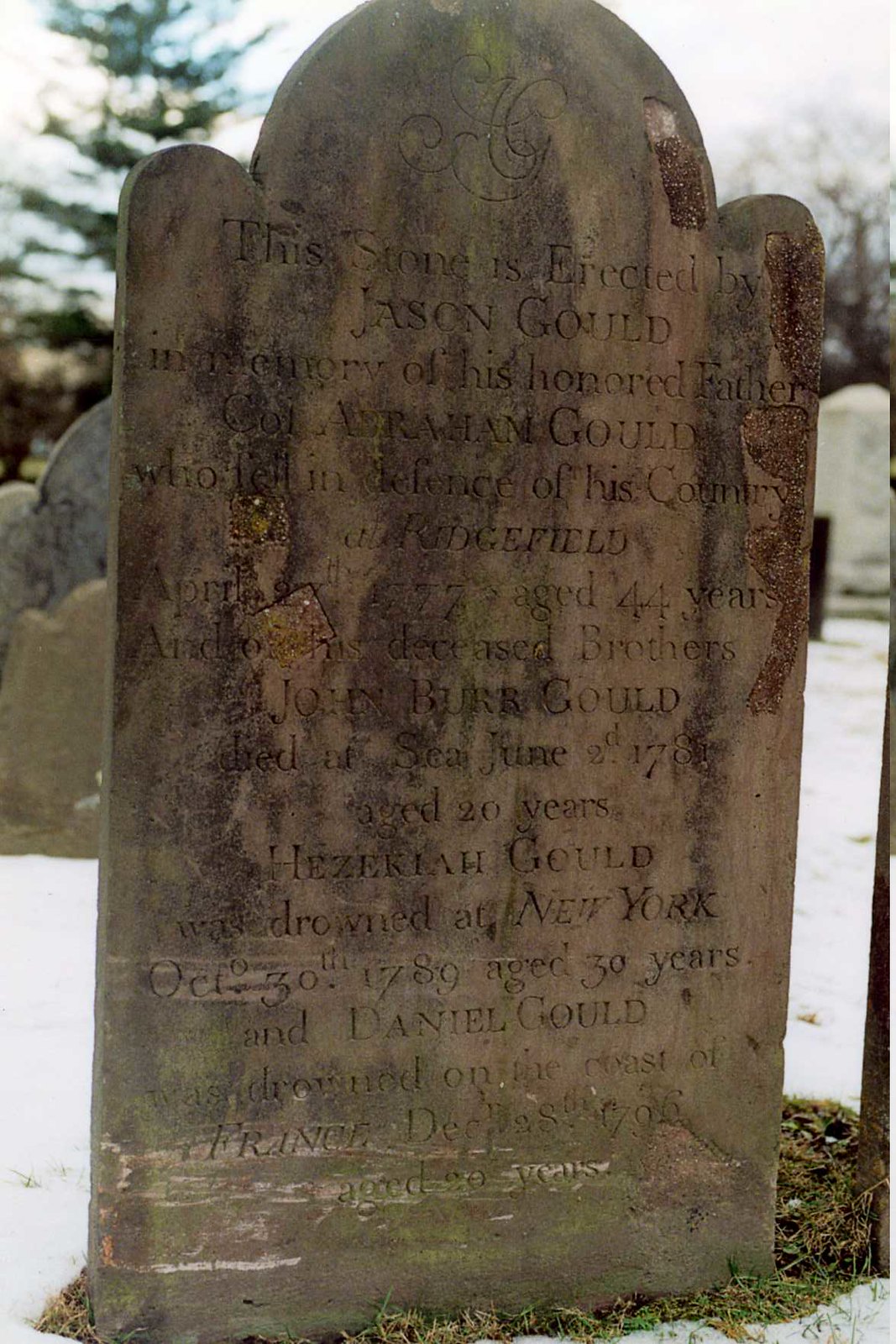The image depicts an aged and weathered gravestone, predominantly rectangular, save for the intricate detailing at its top: two small circles on either side and a prominent half-circle at the very crest. The gravestone stands on a patch of moss, its surface marked by greenish discoloration and patches of moss, indicating its lengthy exposure to the elements. Despite the wear and tear, the inscription reads: “This stone is erected by Jason Gould, in memory of his honored father, Cole A. Raughan Gould, who fell in defense of his country. April 27, 1777, age 44. Andrew, his deceased brothers, John Burr Gould, died at sea June 2, 1781, age 20 years, Hezariah Gould, who drowned at New York October 30, 1789, age 30, and Daniel Gould, who drowned on the coast of France, De Glasse, December 28, 1706, age 20 years.” In the background, blurred trees and other headstones or possibly a mausoleum are visible, adding to the somber and historical ambiance of the scene.